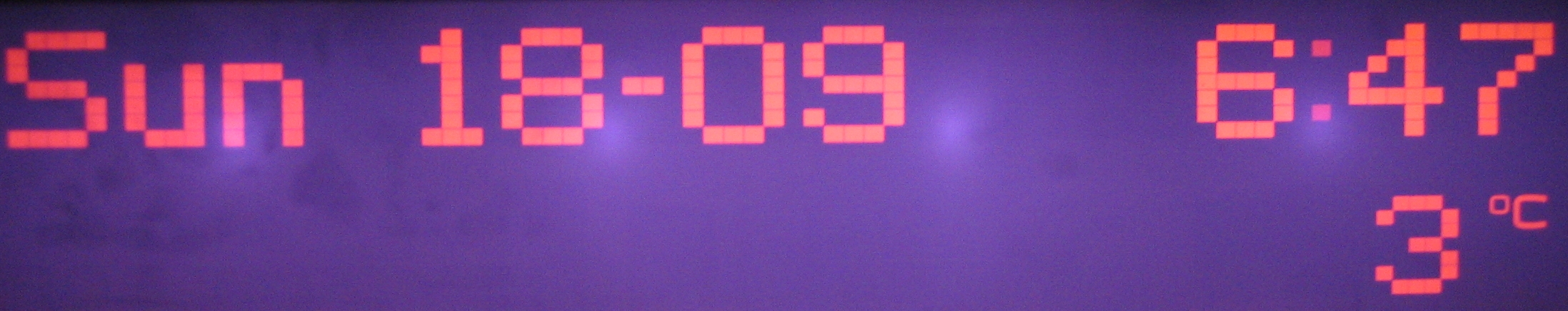The image features a long, sleek digital clock encased in a deep, shiny purple box. The clock displays the day "Sunday," the date "1809," the time "6:47," and the temperature "3°C" in striking red digital letters, composed of numerous connected dots. Measuring approximately 10 inches in length, this modern timepiece emits a soft glow, reflecting off the surrounding wall, with four small lights concentrated in its center, adding a subtle touch of illumination to the scene.